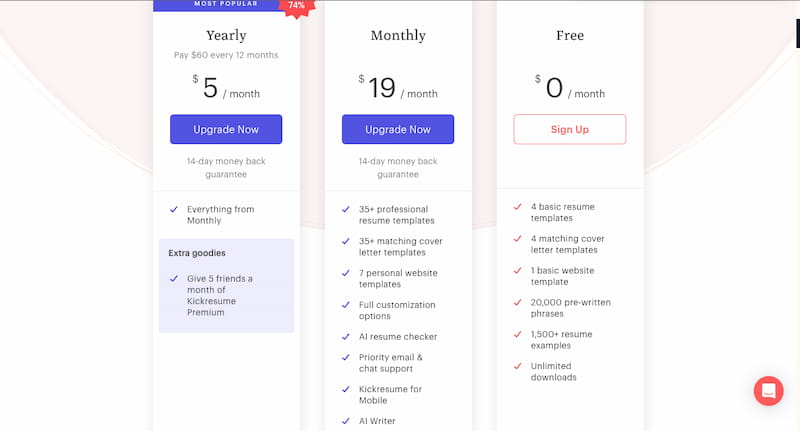The image depicts a subscription plan comparison for a website builder. The basic plan, which costs $5 per month, is the most popular choice and covers essential features. The most comprehensive option is the $19 per month plan, which includes additional tools such as AI capabilities and personal website templates. There is also a free plan available, providing basic resume creation and minimal personal website features, with the option to upgrade for more advanced website functionalities.